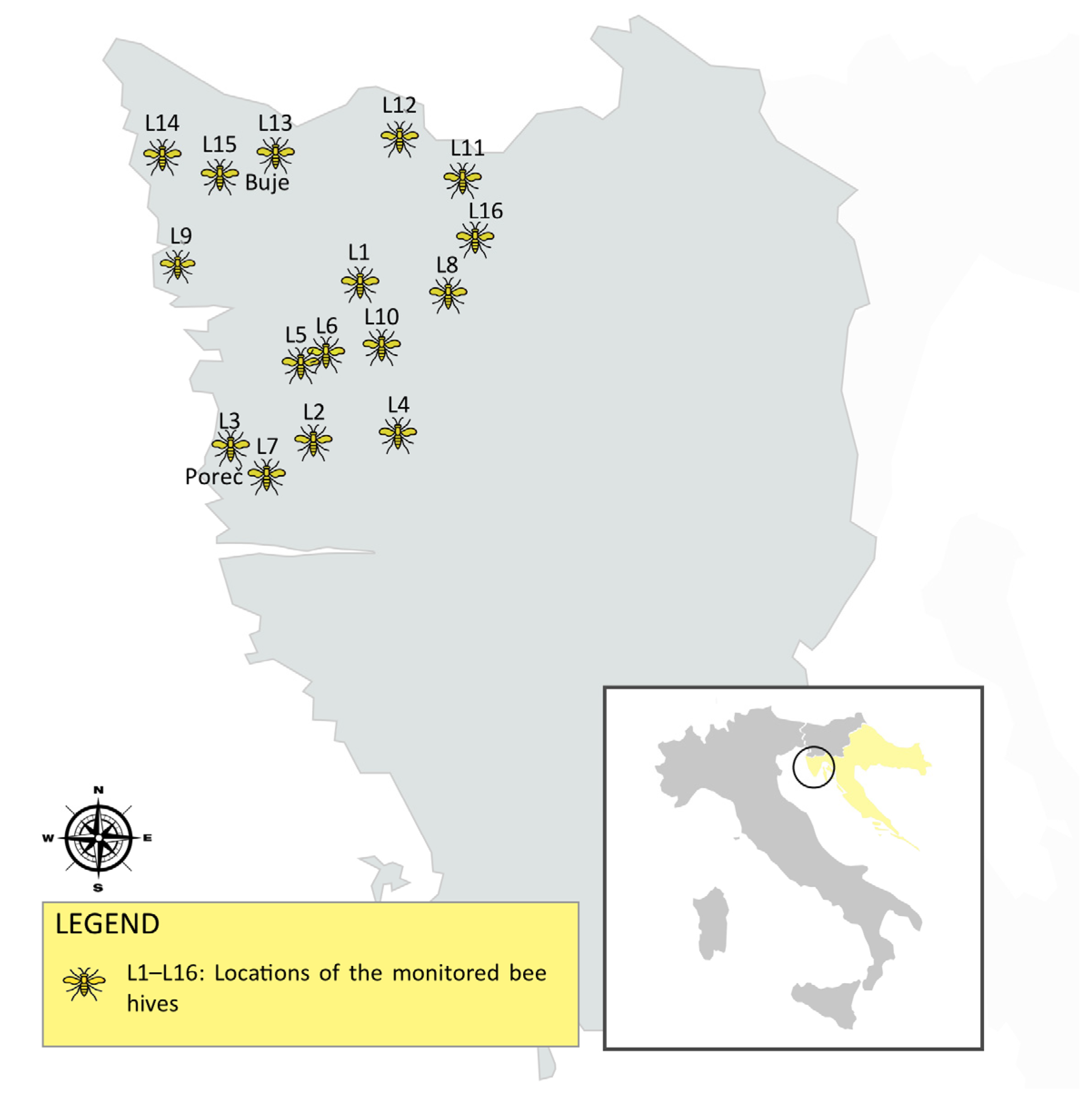This infographic, set against a white background, predominantly features a grey map of a landmass, with the upper left section highlighted in yellow. The primary focus is the monitored beehives across this yellow-highlighted area, each labeled L1-L16. On the bottom right of the infographic, there's an inset showing a broader map that includes Italy and parts of a neighboring country, providing geographical context. The larger map circles the area of focus, which is then magnified on the main map. An adjacent compass is also present, indicating the cardinal directions (north, south, east, west) and a legend in yellow with an illustration of a honeybee. The legend explains that the labels L1-L16 correspond to the locations of these monitored beehives. Specific locations are indicated on the map with the bees scattered primarily across the top left section, each bee's position denoted by its specific label.